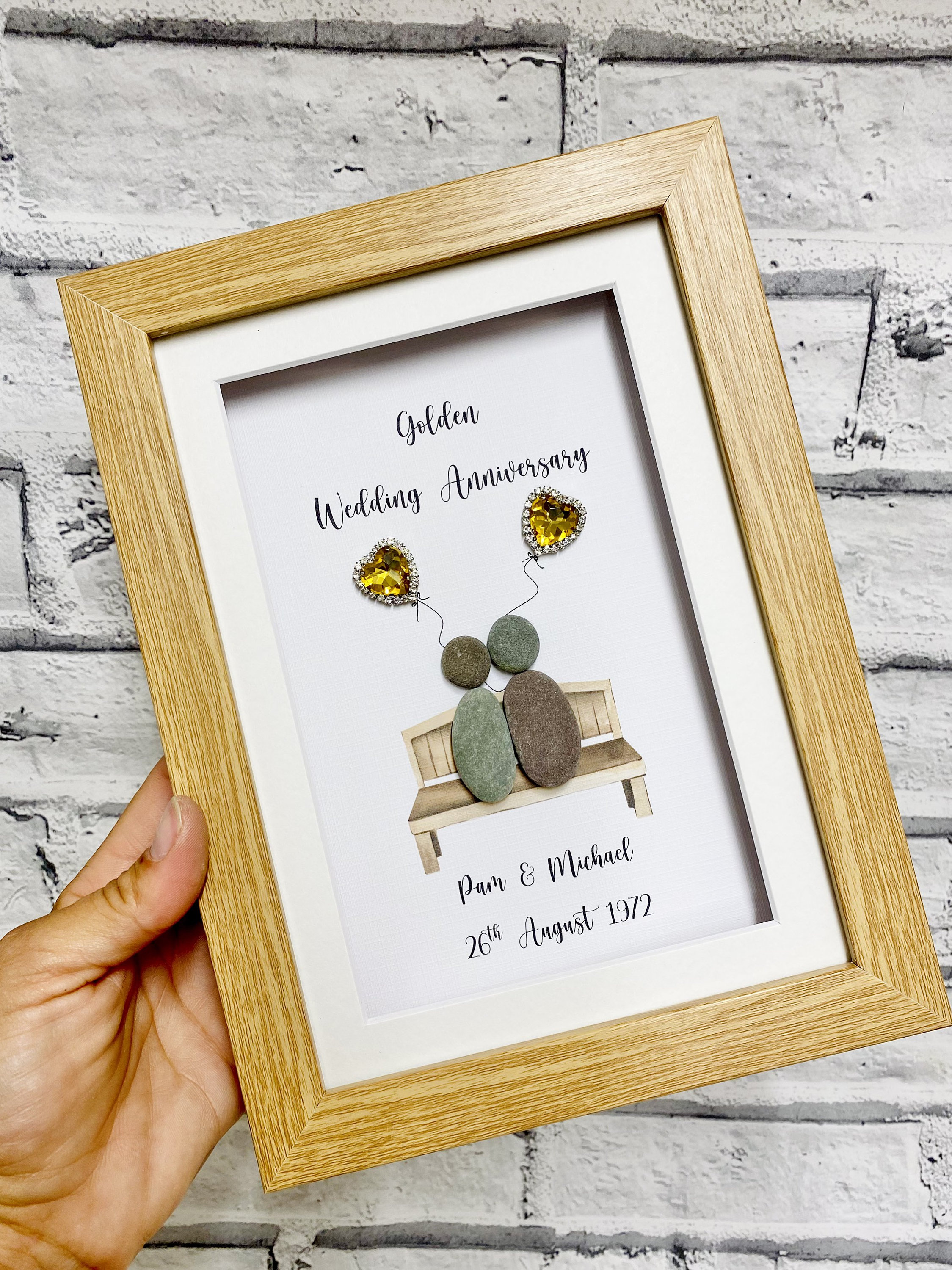In the lower left corner of the image, a Caucasian left hand holds a framed picture against a background of an aged white brick wall. The frame is made of light-colored wood with a white mat surrounding the artwork. The picture itself features the black ink inscription: "Golden Wedding Anniversary, Pam & Michael, 26 August 1972." Central to the artwork is a bench with two abstract figures made of stones; the figure on the left has a brown circular head and a greenish oblong body, while the figure on the right has these colors reversed. Above these figures float two heart-shaped balloons made of topaz-colored gemstones, outlined with small rhinestones and attached to drawn string lines to complete the balloon effect.